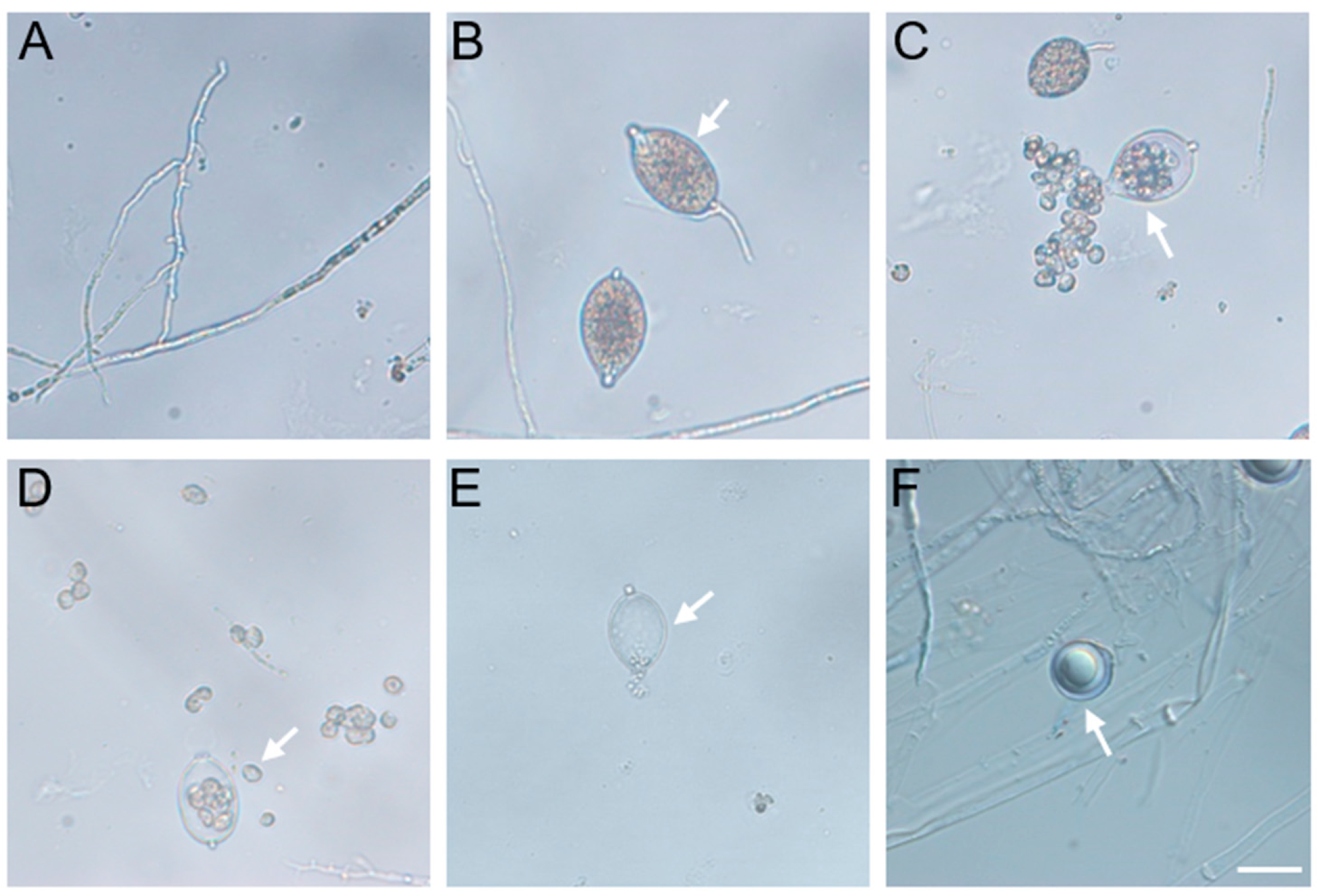The image consists of six microscope slides, labelled A, B, C, D, E, and F, arranged in two rows of three. Slide A features a network of linear structures, reminiscent of cracked glass or small rivulets, with clear central regions and bluish hues along the sides. Slide B showcases two ovate shapes with speckles, primarily brown with a light gray background. One of the ovate shapes has a distinct white tail and is highlighted with a white arrow. Slide C presents a ruptured ovate form releasing numerous small, bubble-like structures, outlined in light blue with peach-colored interiors, also indicated by an arrow. Slide D continues the theme with fewer bubbles contained within a blobby structure. Slide E displays a see-through oval shape devoid of internal bubbles, while Slide F depicts a raised, pimple-like circle with a surrounding ring. Arrows throughout the slides guide the viewer's focus to specific details within the microscopic views.